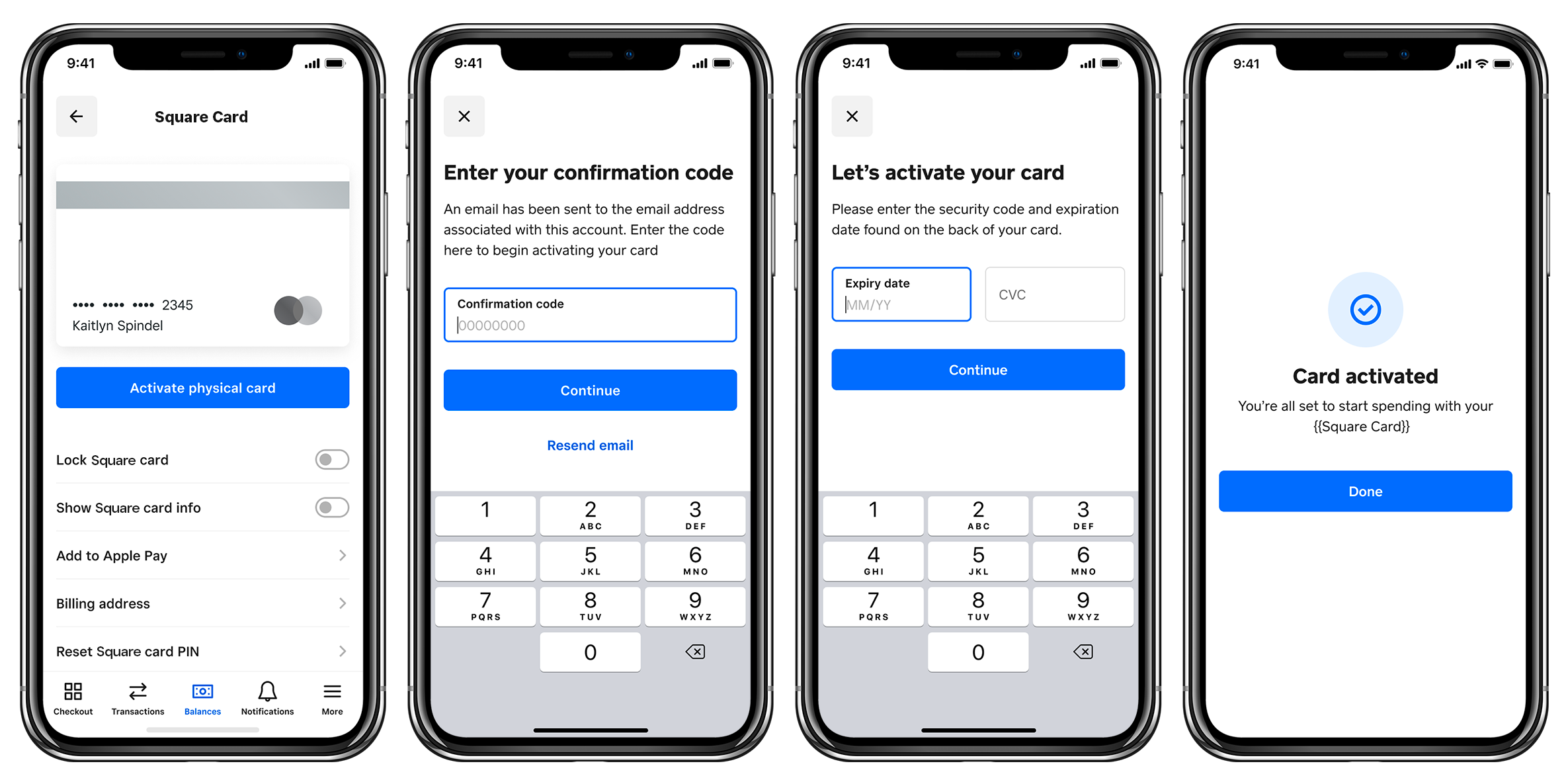The image displays four identical cell phones oriented face-up, each presented in various shades of gray. Despite their identical looks, each screen showcases distinct content while featuring common elements - a prominent blue rectangular button set against a white background.

The phone in the upper left-hand corner depicts detailed financial or transactional information. The screen first displays the value "941 per ton," along with connectivity indicators showing four signal bars and a full battery icon. Below this, there is a gray box with an arrow pointing to the left, labeled "square card."

Following this, a section shows a sequence of four horizontal dots, a space, another set of four horizontal dots, a space, another set of four horizontal dots, another space, followed by five more dots. To the right of these dots, there is a gray slider. Directly beneath this sequence, the name "Caitlin Spiedel" is displayed.

The blue rectangular button on this screen reads "Activate Physical Card". Below it, there are additional options: "Lock Square Card" with a slider to the right, "Show Square Card Info" with a slider to the right, "Add to Apple Pay" with a right-pointing arrow, "Billing Address" with a right-pointing arrow, and "Reset Square Card PIN" also indicated with a right-pointing arrow.

At the bottom of the screen, there are five icons resembling typical menu options, possibly labeled as follows: "Checkout", "Transactions", "Resources", "Notifications", and "More".